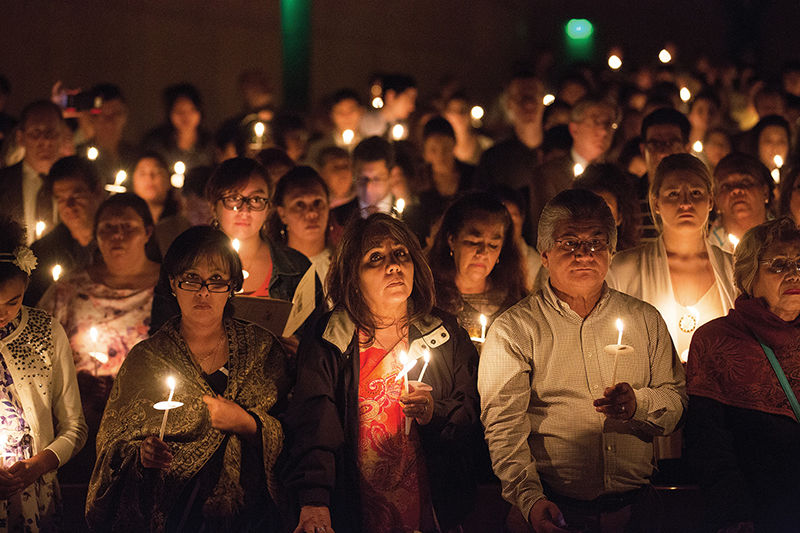The photograph is a vivid and dramatic night shot capturing a large group of solemn individuals participating in what appears to be a vigil. The image is taken in landscape orientation, approximately six inches wide and three to four inches high, with a focused foreground and a gradually blurring background. The front row features a few middle-aged women, an elderly man, and an elderly woman, all with similar dark complexions, thick hair, and somber expressions, suggesting they might be related. Each person is holding a thin white lit candle with a brown paper wax catcher. The entire scene is illuminated by the soft, warm glow of the candles, casting a brownish tint over the participants and enhancing the serious mood. In the backdrop, a brown wall is faintly visible, along with a green light on the right-hand side and a vertical gap on the upper left. The crowd extends deep into the image, implying a large turnout, with people standing very still, their solemn faces either looking towards the camera or downward in reflection. An indistinct, possibly blurry cell phone can be spotted on the upper left, further adding to the somber atmosphere of this contemplative gathering.